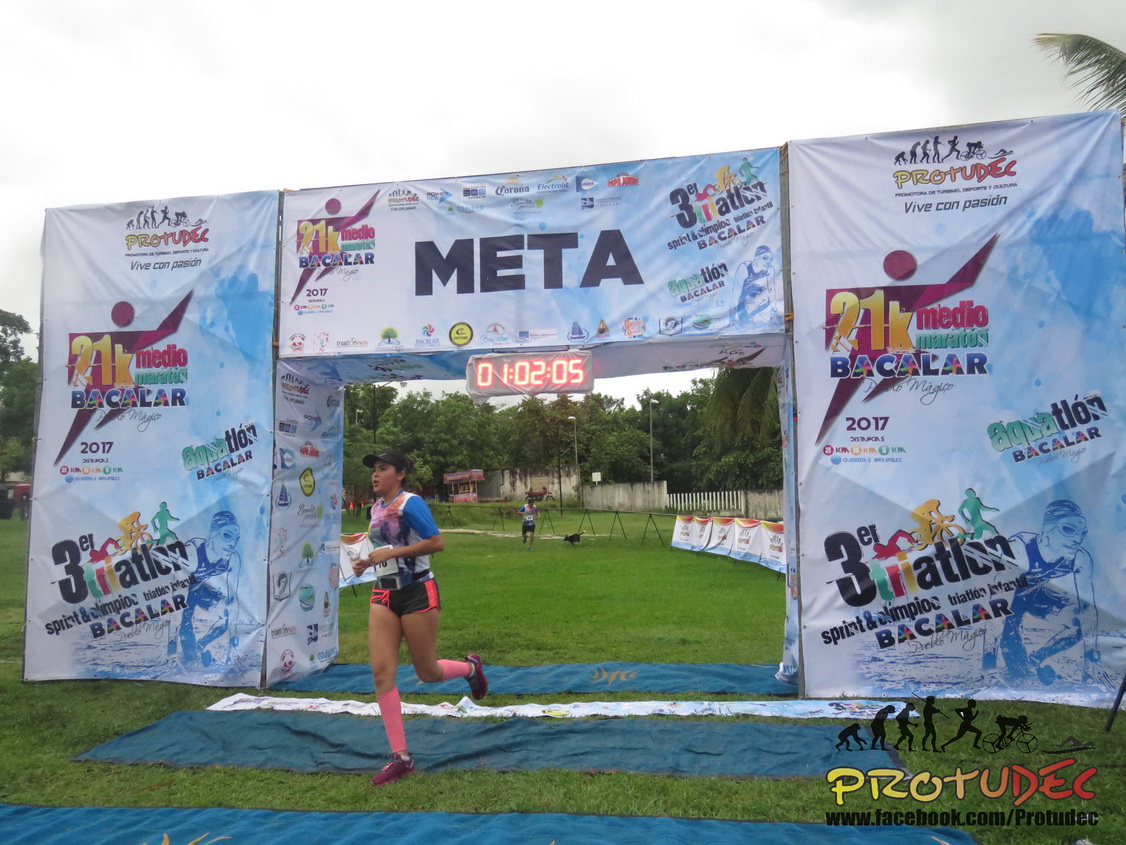The image depicts the finish line of a race set against a large grassy field, with a blue sky overhead and a wooded area featuring a white picket fence in the background. Central to the image is an archway bearing the text "META" at its top, with an elapsed time of 01:02:05 displayed beneath. A single female runner, dressed in a blue jersey, black shorts with pink stripes, and pink socks and running shoes, is crossing the finish line at the center of the frame. Blue mats with a white stripe mark the finish line on the grass. The runner wears a race bib on her jersey, indicating her number. The lower right corner of the image features text in red and yellow, likely "ProDetect,” possibly the name of the organizing company. Advertisements for "Third Nation Spirit" and "Champion Bacalar" are visible on one side of the archway. No other runners are in sight, hinting that the woman may be leading the race. A person stands with a dog in the background, possibly observing or photographing the event. The scene suggests a daytime setting during a marathon, half marathon, or triathlon event.